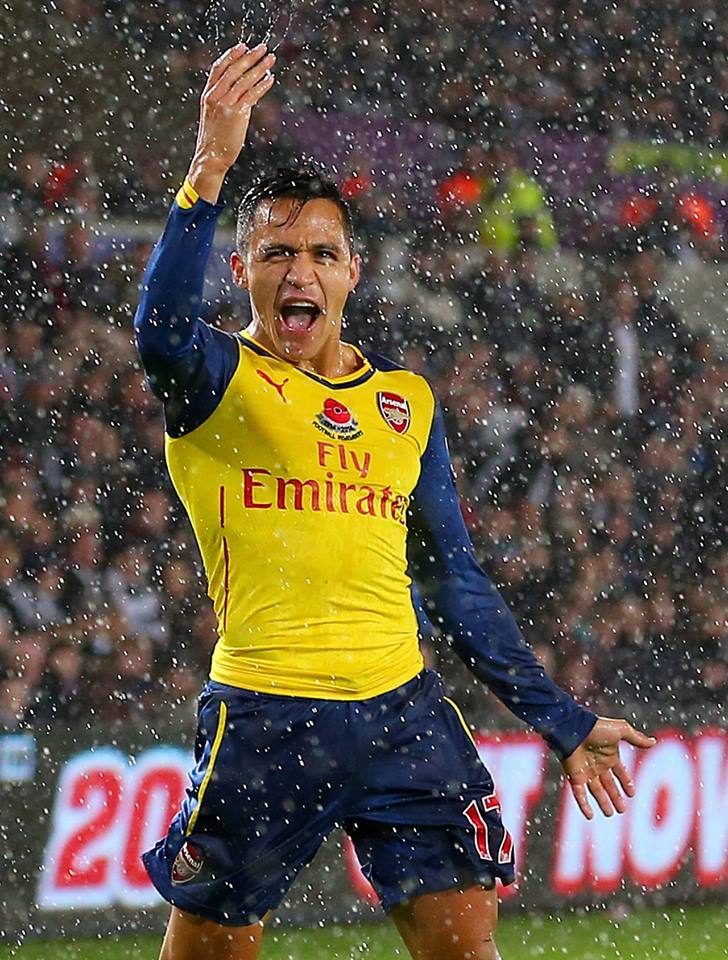In the photograph, a male soccer player stands on a rain-soaked field during the daytime, completely drenched from head to toe. His jersey is a striking combination of blue long sleeves and a yellow center, emblazoned with "Fly Emirates" in red. A distinctive emblem resembling a Pokeball and a red shield with white, unreadable text adorn the left side of his jersey. He sports blue shorts with a yellow stripe down the side, marked with the number 17. 

The athlete's black hair is slick with rain, and water droplets cascade off his raised right hand. His mouth is agape as he gazes straight ahead, seemingly in the midst of an ecstatic moment, possibly having just scored. The grass field beneath him is visible, emphasizing the outdoor setting.

In the blurry background, a packed stadium crowd watches intently. A large red "20" outlined in white is clearly visible on a banner behind him, along with the partial words "NOW" and "November." Advertisements and various colors in the audience add to the vibrant, chaotic atmosphere. The entire scene is speckled with raindrops, giving the image a dynamic and energetic feel.